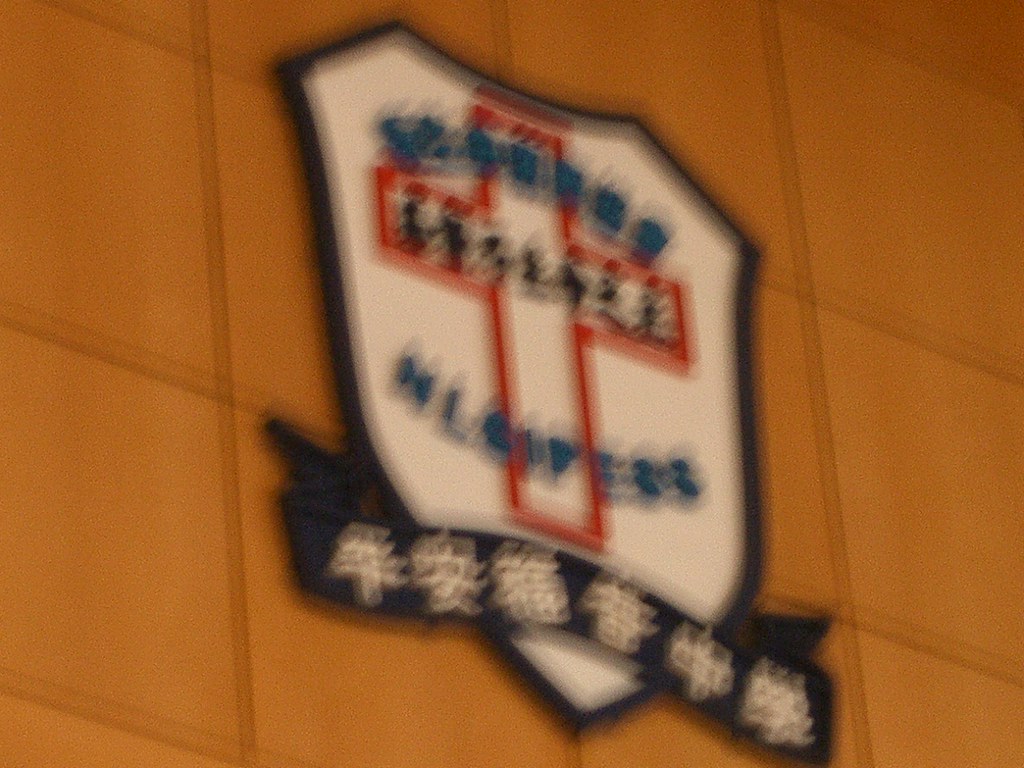This image depicts a somewhat blurry crest mounted on a brown wall. The crest features a predominantly white background with detailed accents in blue, red, and navy blue. Central to the design is a prominent red cross, reminiscent of the symbol used by the Red Cross organization, though it’s unclear if it has any formal association. The crest incorporates text written in blue, but the blurriness renders the words illegible. Notably, there are foreign characters at the bottom, possibly of Asian origin, suggesting an international context or affiliation. While the exact significance of the crest remains ambiguous due to the blur, its detailed elements hint at a meaningful emblematic design.